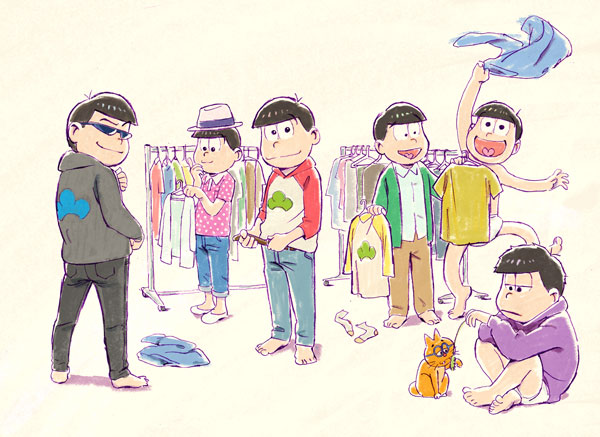This is a detailed pixel art illustration depicting five kids in a clothing store, all rendered in the same distinct, simplistic style with flat bangs and large, white cartoon eyes, typical of a certain cartoon aesthetic. They all have vaguely Asian features and are engaged in various activities surrounding trying on different clothes. Behind them, two racks of clothing on hangers set the scene in the store.

Starting from the left, the first child is wearing sunglasses, a dark grey hoodie, and black pants, with his back turned slightly but head facing the viewer. Next to him, another child is sporting a pink and purple fedora, a white and pink polka dot polo shirt, and blue capris, clearly in the midst of another outfit experiment. Another kid towards the center is putting on a brown belt over a white and red hoodie paired with blue pants, absorbed in his task.

A striking figure near the middle-right appears in just his underwear, energetically waving his pants around his head with a wide, playful expression. Meanwhile, on the far right, a child in underpants sits on the floor wearing a purple hoodie, entertaining a cat on a leash. The cat, notable for its tiny sunglasses, adds a whimsical touch to the scene.

In the background, additional clothing racks illustrate the store setting, reinforcing that these kids are exploring various fashion choices in a lively, shared space.